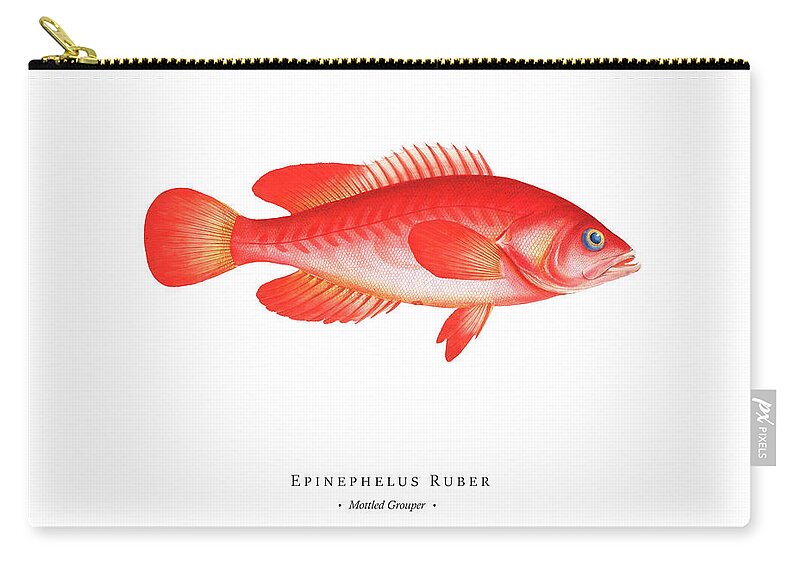This image features a detailed, white handbag, likely made of leather or canvas, that could be sold on a website or displayed in an aquarium gift shop. The handbag is characterized by a golden zipper at the top, complemented by a black lining. The zipper appears to be on the left, suggesting either an open or closed state depending on the viewer’s interpretation. Across the front center of the bag, there is a vivid illustration of a red-orange fish, identified as a modeled grouper, or scientifically as "Epinephelus ruber." The fish’s intricate details include a fin on the top and bottom, two side fins, a tail reminiscent of a paintbrush tip, and subtle yellow accents on its fins and tail base. The pencil case or art supply bag also features a gray rectangular tag at the bottom right corner, labeled with "PX pixels" in white text, adding a modern touch to its classic scientific illustration theme.